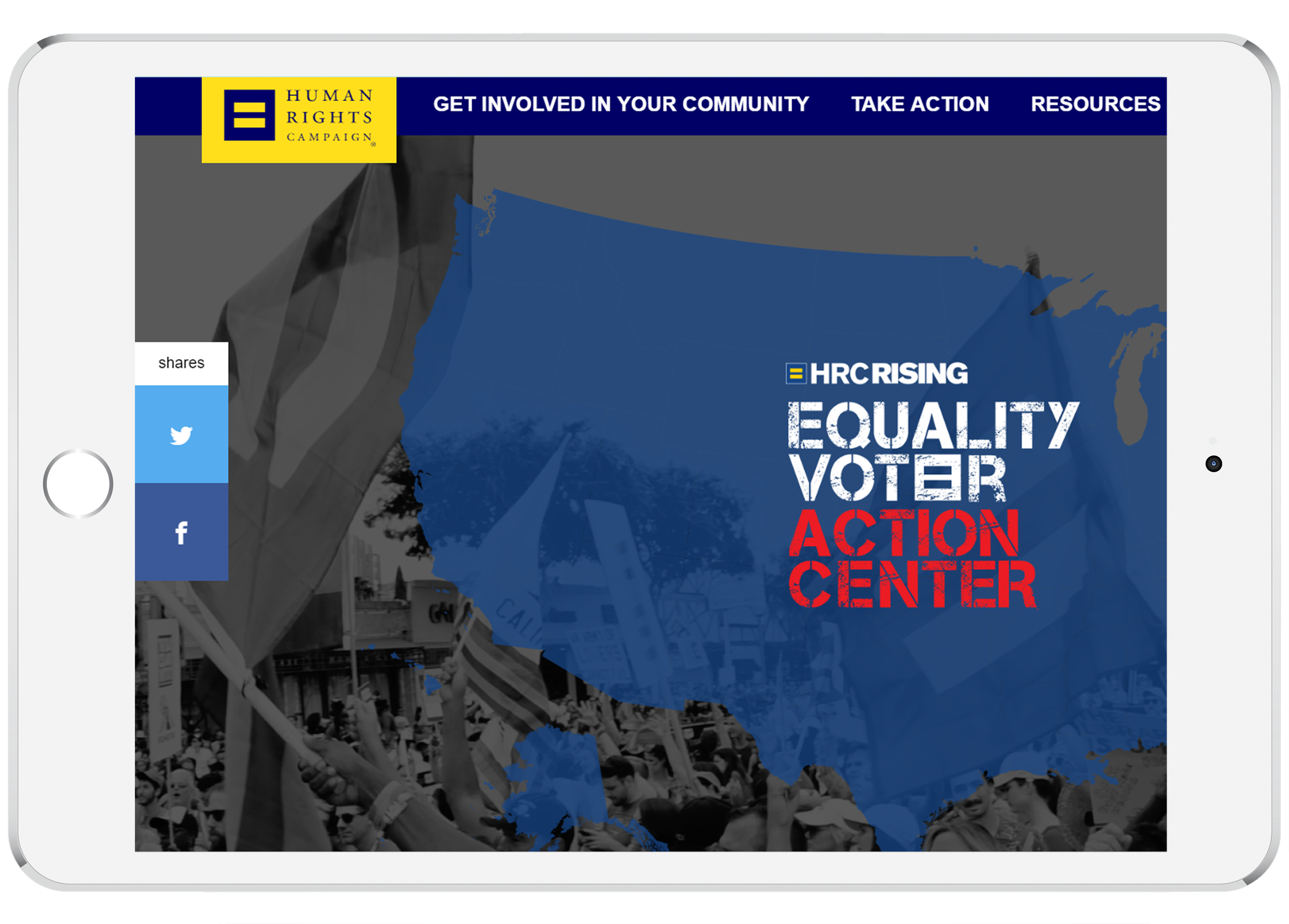The image features a white iPad turned sideways, displaying content from the Human Rights Campaign. The iPad screen shows a vibrant yellow square containing a blue square, which holds a yellow equal sign, recognizable as the Human Rights Campaign logo. At the top of the screen, menu options read: "Get involved in your community," "Take action," and "Resources." On the left side, social sharing icons for Twitter and Facebook are visible.

The background of the iPad screen displays a black-and-white image of a protest with numerous indistinct figures holding various flags, framed by city buildings. An opaque blue outline of the United States is superimposed over this scene, highlighting the words "HRC Rising Equality Voter Action Center."

The iPad itself is distinctly visible, characterized by its white border. The home button is located on the left edge of the image, and the front-facing camera is positioned on the right edge, corresponding to the device's landscape orientation.